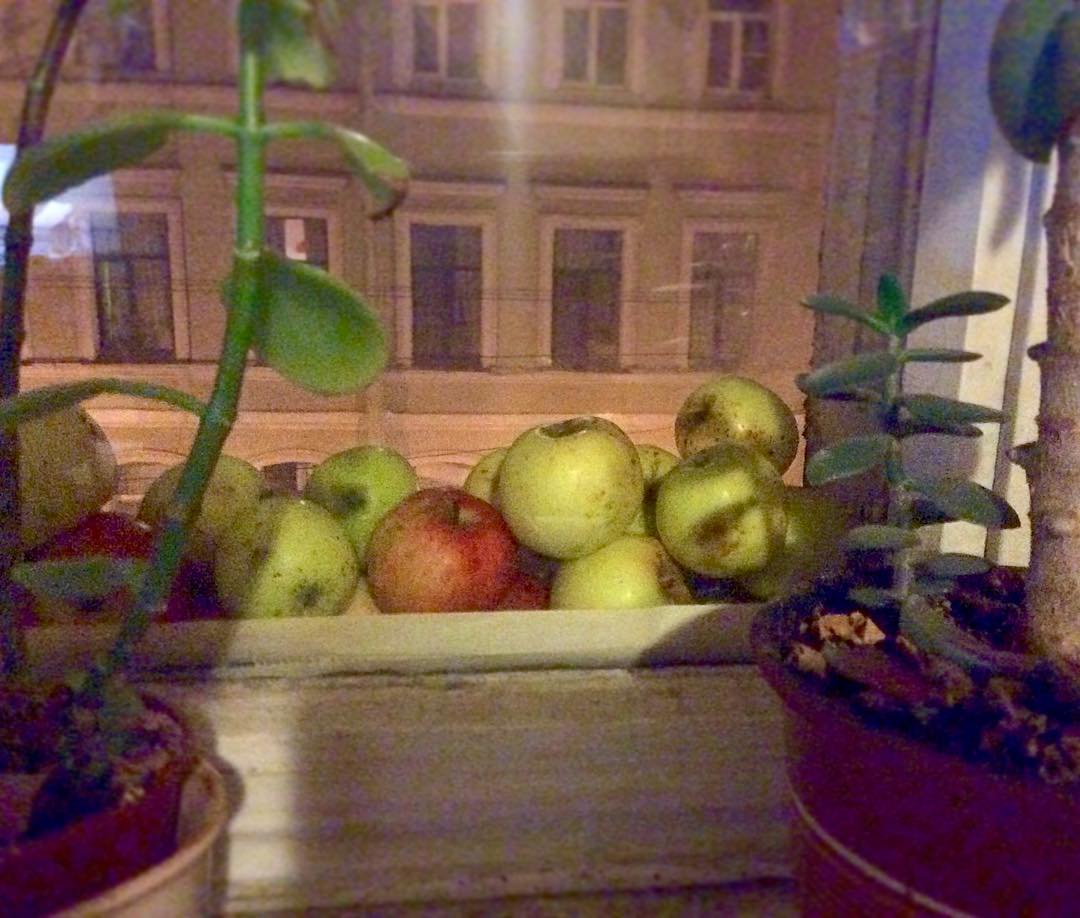This photograph, presented as a horizontal rectangle, captures a dimly lit, grainy scene of an urban apartment windowsill. The inside window frame, painted white, envelops a wooden ledge supporting an assortment of items. In the foreground, there are two potted plants—one on the left with a white outer pot containing a red pot with a tall green plant, and one on the right with a red pot. This right-side plant splits into two varieties: one with green stems and leaves, and another with a woody brown stem leading to green leaves.

Scattered across the windowsill are roughly 12 apples in varying hues, including around 10 green apples and a few red ones. The window offers a view of an exterior building, identifiable by its white and cream-colored facade and several darkened windows arranged in visible rows. The building’s many windows, adorned with white curtains, suggest an urban environment. The scene outside appears to be nighttime, with the positioning of the camera indicating the photo was taken from a fairly elevated floor, providing a close, detailed look into the apartment’s cozy yet cluttered windowsill.